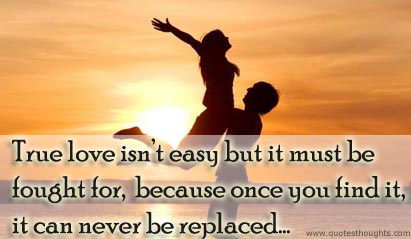The image captures a stunning beach landscape at sunset, with a brilliant orange sky and the sun partially obscured by clouds, casting a reflection on the muddy waters of the shoreline. At the heart of the scene, silhouetted against the glowing backdrop, a man stands on the right, lifting a woman high. The woman, positioned to the left, has her arms wide open and legs stretched out behind her, reminiscent of the iconic lift from "Dirty Dancing." Her long hair flows as she leans back, both figures appearing as dark shadows framed by the radiant light. Across the bottom of the image, bold black text reads, "True love isn't easy, but it must be fought for, because once you find it, it can never be replaced..." In the bottom right corner, in very small font, is the website URL www.quotesthoughts.com. The text is set against a semi-transparent white background that spans the lower portion of the image, ensuring the quote stands out clearly.